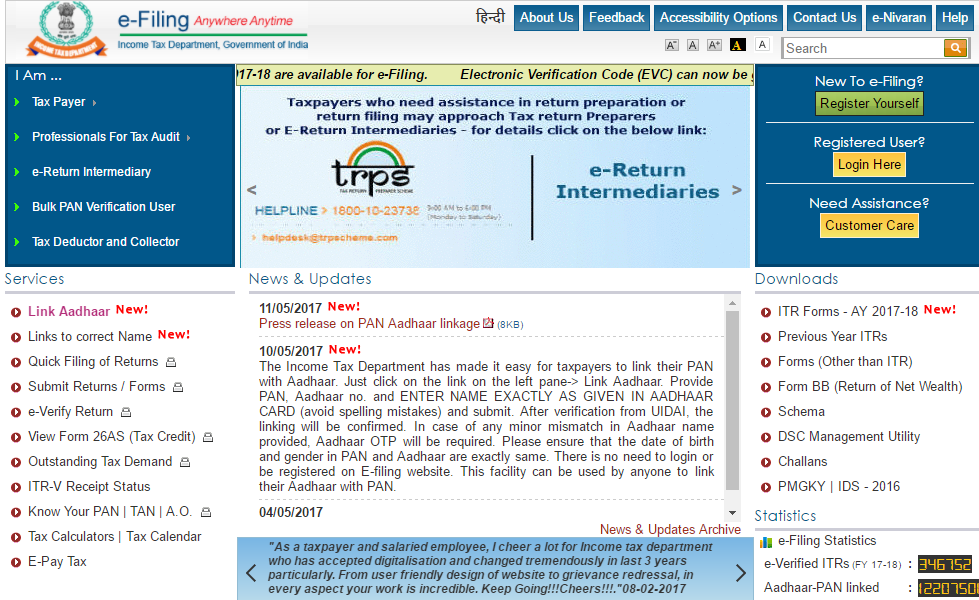The image depicts a webpage from the Income Tax Department of the Government of India’s e-filing portal. At the top, it prominently displays the words "e-Filing: Look Anywhere, Anytime." On the right side of the page, there is a menu that includes options such as "About Us," "Feedback," "Accessibility Options," "Contact Us," "e-Nivaran," and "Help." A search bar is also located on the right.

Central to the image is a blue box containing various user options, including "I am a taxpayer," "Professional for Tax Audit," "e-Return Intermediary," "e-PIN Verification User," and "Tax Deductor and Collector." Within this blue box, a light blue section provides information about Tax Return Preparers (TRPs). It states that taxpayers needing assistance with return preparation or filing can approach TRPs and mentions "e-Return Intermediaries."

On the right-hand side of the image, there is a date stamp of 15th November 2017, alongside a note about a new press release on linking PAN with Aadhaar. Additionally, there's information dated 5th October 2017, detailing how the Income Tax Department has simplified the PAN-Aadhaar linkage process, including instructions on how to complete it.

Towards the bottom, another blue box contains links specifically aimed at taxpayers and salaried employees. On the left side of the page, there are various helpful links, while the right side offers a range of downloadable resources.